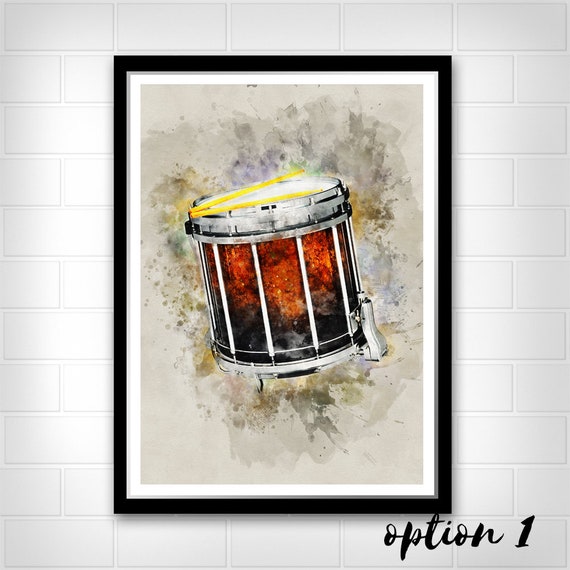The image depicts a framed piece of wall art featuring a stylized depiction of a snare drum. The artwork is mounted on a white brick wall and is presented within a black frame. The snare drum, with vertical white strips and a silver rim at both the top and bottom, is set against a light grayish-beige background that is artfully splattered with watercolor splotches in shades of gray, brown, purple, and green. Accentuating the drum are two yellow drumsticks resting across its top. The watercolor effect behind the drum gives the impression of movement and sound, with abstract splashes enhancing the visual dynamism. Additionally, the bottom left corner of the artwork features the handwritten script "option one."